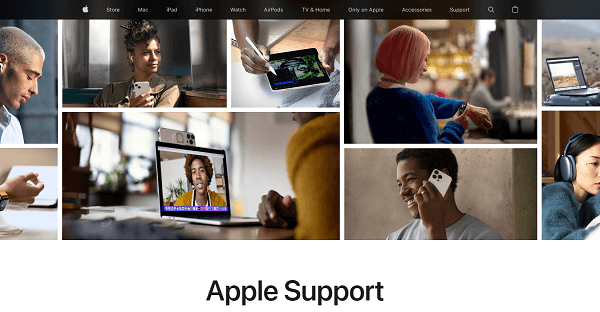This is an image capture of an Apple website homepage. At the very top, there is a black navigation bar with a variety of clickable options, about seven in total, including icons for sharing and a magnifying glass for search functionality. Below this navigation bar are images featuring a diverse group of individuals from different backgrounds, all engaged with Apple products, such as computers, laptops, tablets, and phones. Underneath these images, there is a section labeled "Apple Support." Interestingly, the individuals depicted seem to be predominantly from minority groups, with possibly one person who could be Caucasian, highlighting Apple's effort to showcase diversity. Despite seeking support, all the individuals appear to be in a positive, happy demeanor. The overall layout aims to provide easy access to support while emphasizing a diverse and content user base.